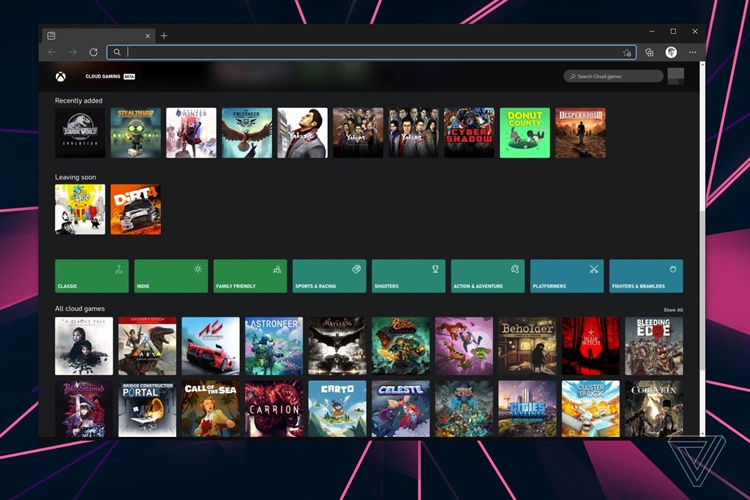The image displays a desktop screenshot with an abstract neon purple and pink light design as the background. Open on the screen is a web browser showcasing the Xbox Cloud Gaming beta interface. The 'Recently Added' section includes games such as a Jurassic Park-themed game, a title that resembles "Philisteel," "Frontier Winter," "The Falconeer," two or three Yakuza series games, "Cyber Shadow," "Donut County," "Desperados III," and "Dirt."

Several categories are listed for ease of navigation, including 'Classic,' 'Indie,' 'Family-Friendly,' 'Sports & Racing,' 'Shooters,' 'Action Adventure,' 'Platformers,' 'Fighters & Brawlers.' Game titles visible in the image include "Ark," a car racing game, "The Last Roaner," which might be related to Batman, "Beholder," "Blair Witch," "Bleeding Edge," "Portal," "Call of the Sea," "Carrion," "Cardo," "Celeste," "Cluster Truck," and several others that are difficult to read. The overall screen depicts an organized and vibrant gaming catalog, albeit with some text too small to decipher accurately.